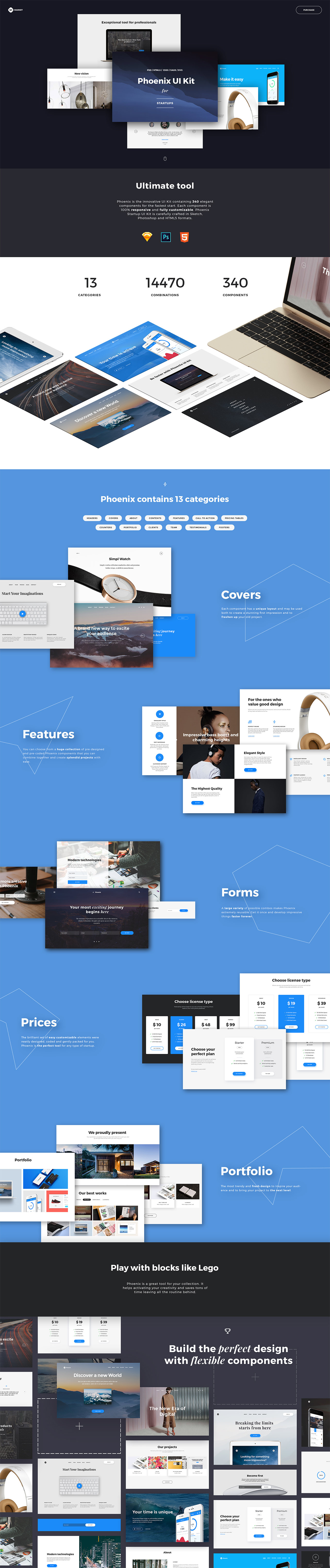[Phoenix UI Kit Advertisement]

The advertisement is a long, rectangular screenshot designed to showcase the Phoenix UI Kit. Let's break down the contents, section by section, for a detailed description:

**Top Section:**
- **Background:** Dark black
- **Content:** Features six images:
1. **Hanging Pans:** Image showing assorted pans hung on a rack.
2. **Laptop:** Image of a laptop displaying a black screen with white writing.
3. **Cell Phone Settings:** Image of a cell phone against a blue background, displaying a settings page with a white screen and a blue circle.
4. **Headphones:** Image of white headphones with tan ear pads.
5. **People's Faces:** Image on a white background with three circles showing people's faces along with some text.
6. **Phoenix UI Kit:** Image with a dark blue background and varying dark blue wave shades, prominently displaying the text "Phoenix UI Kit."

**Subheader:**
- **Background:** Black bar
- **Content:** Text reads "Ultimate Tool," followed by a paragraph that is too small to make out, and includes three symbols: 
  1. **Yellow Diamond:** Icon of a yellow diamond.
  2. **PS Box:** Icon of a box with "PS" written inside.
  3. **Red Shape:** Icon with the number "5" inside a red shape.

**Second Section:**
- **Background:** White
- **Content:**
  - Text readings: "13 categories," "14,470 combinations," and "340 components."
  - Visuals: 
    - A laptop is displayed on the right side.
    - Six flat screens/pages laid out:
      1. One depicting a road.
      2. One showing cell phones.
      3. One displaying a laptop.
      4. One with a black background and white text.
      5. One featuring a mountain range at sunset.

**Main Section:**
- **Background:** Blue
- **Content:**
  - Header Text: "Phoenix contains 13 categories."
  - Categories: Displayed in small, white oval tabs (too small to read specifically).
  - Various images:
    - A white keyboard.
    - A watch with a black band and gold rim.
    - A snow-capped mountain range.
  - Right side text: "Covers" with some accompanying text.
  - Features Section: Depicts four images:
    - White headphones.
    - Two images of people wearing headphones.
    - Several circles with accompanying text.
  - Forms Section: Located on the right, with associated writing.
    - Images include:
      1. A table leg.
      2. A person bent over a table with pictures in front of them.
  - Prices Section: Displays four images with different colored boxes (blue, white, and gray) and various prices ($10, $30).
    - Text: "Choose your perfect plan."

**Portfolio Section:**
- **Right side text:** "Portfolio."
- **Content:**
  - Four images featuring various scenes:
    - A laptop.
    - Keyboards and screens.
    - A house with garage doors.
    - Cell phones.

**Bottom Section:**
- **Background:** Black
- **Content:** 
  - Text reads "Play with blocks like Legos" and "Build the perfect design with flexible components."
  - Several white boxes with text and cropping tools.

This detailed description provides a clear and structured overview of the advertisement's layout, images, and text content.